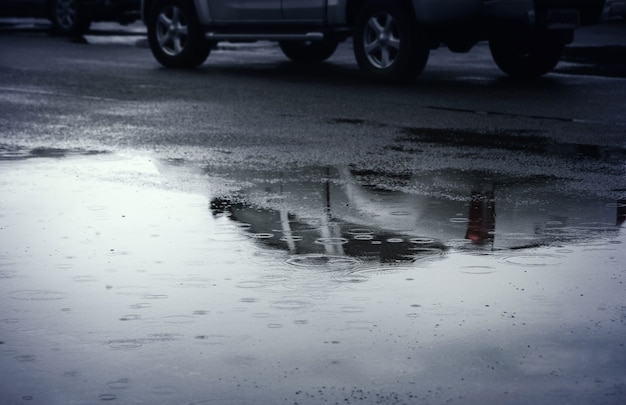The black-and-white photograph captures a dreary, rainy day, focusing on a wet roadway or parking lot. The foreground is dominated by a large puddle spanning the entire bottom half of the image, with visible ripples and small splashes created by ongoing raindrops. The reflections in the puddle reveal the gray, overcast sky and the partial silhouette of a nearby vehicle. Only the bottom portion of the vehicle is visible, specifically its silver, five-spoked wheels and lower side skirts. Scattered pebbles and a small curb add to the texture of the wet asphalt surface. The scene exudes a somber, gray atmosphere, with the landscape and the reflective surface of the puddle emphasizing the continuing rainfall.